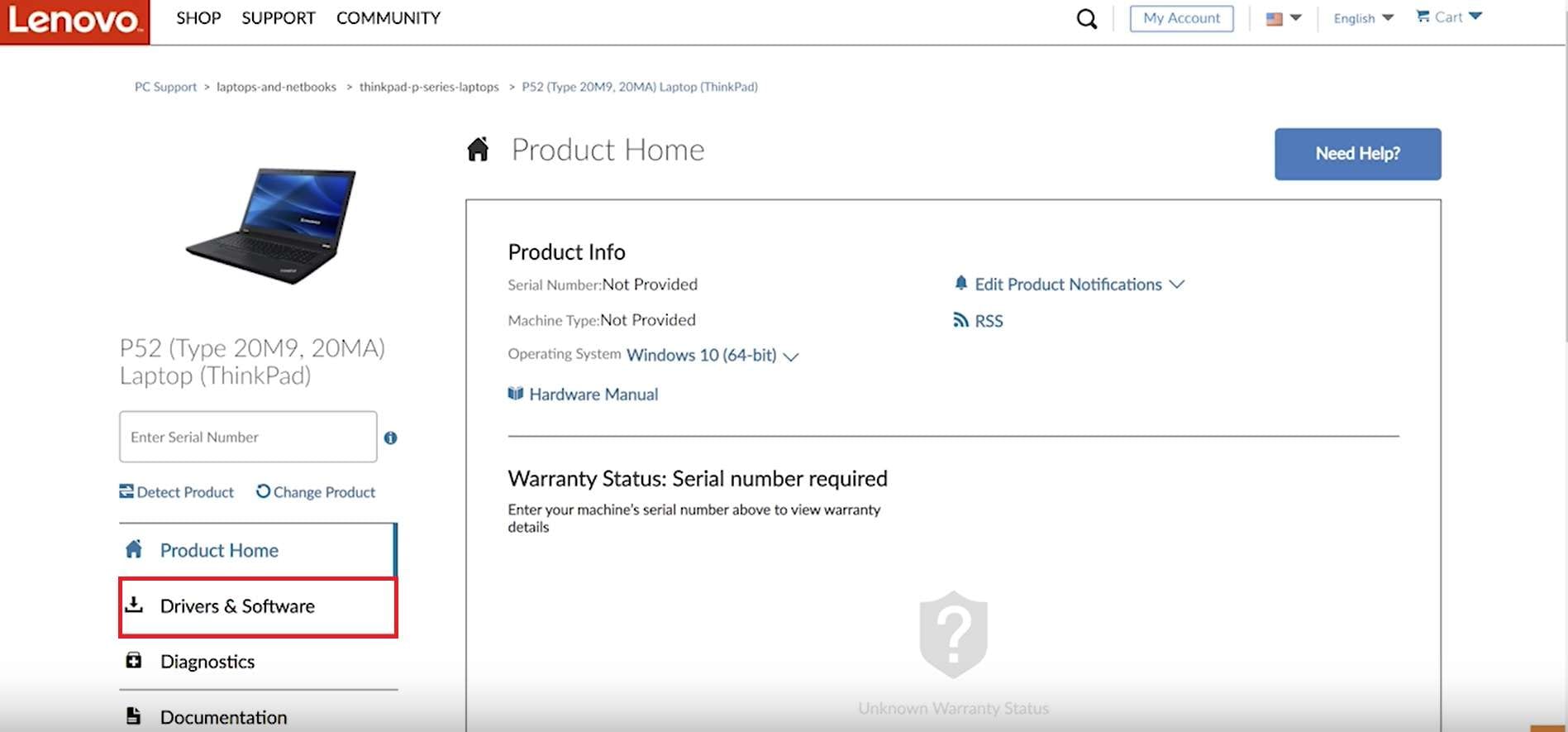This image captures a webpage from Lenovo's website, prominently featuring their branding and navigation elements. On the left side, the word "Lenovo" is displayed in white against an orange-red background. To the right, black text lists navigation options: "Shop," "Support," and "Community." Adjacent to these is a small spyglass icon, and further right, the phrase "My Account" appears in blue. Next to this is an American flag icon labeled "English," followed by a "Cart" icon with a downward-pointing arrow.

Below this navigation bar, the page highlights a specific laptop model: "P5-2 Type 20M9-20MA," belonging to the ThinkPad series. An image of the laptop shows its black and blue design. To the left of the laptop image, "Product Home" is listed, while along the right side is a blue button labeled "Need Help."

Further down, in black text, the product information section reads: "Serial Number Not Provided," "Machine Type Not Provided," and details the operating system as "Windows 10 64-bit." Additional options in blue text include "Edit Product Notifications" and "RSS." Below these, "Hardware Manual" is mentioned. This comprehensive layout aims to provide users with pertinent details and support for purchasing and understanding their Lenovo laptops.